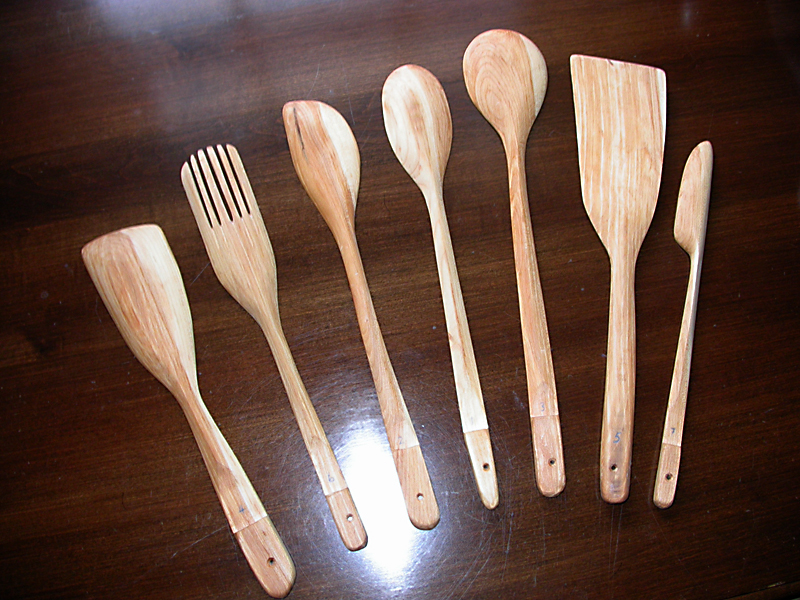This image features a collection of seven wooden kitchen utensils laid out flat on a scratched, brown hardwood table. Photographed from above, the utensils include a variety of shapes and sizes: starting from the left, there's a stirrer, followed by a fork-like tool, then three spoons each differing in shape—one with a shorter, wider oval top, another more elongated oval top, and a third with a rounded top. The utensils continue with a flat spatula and end with a curved spoon. Each tool has a hole in its handle for hanging, and they are all crafted from light-colored wood. A reflected light spot is visible near the fork and third spoon, adding a gleam to the middle of the composition. The utensils are numbered somewhat arbitrarily as 4, 6, 2, 1, 3, 5, and 7, creating an eclectic yet organized display.